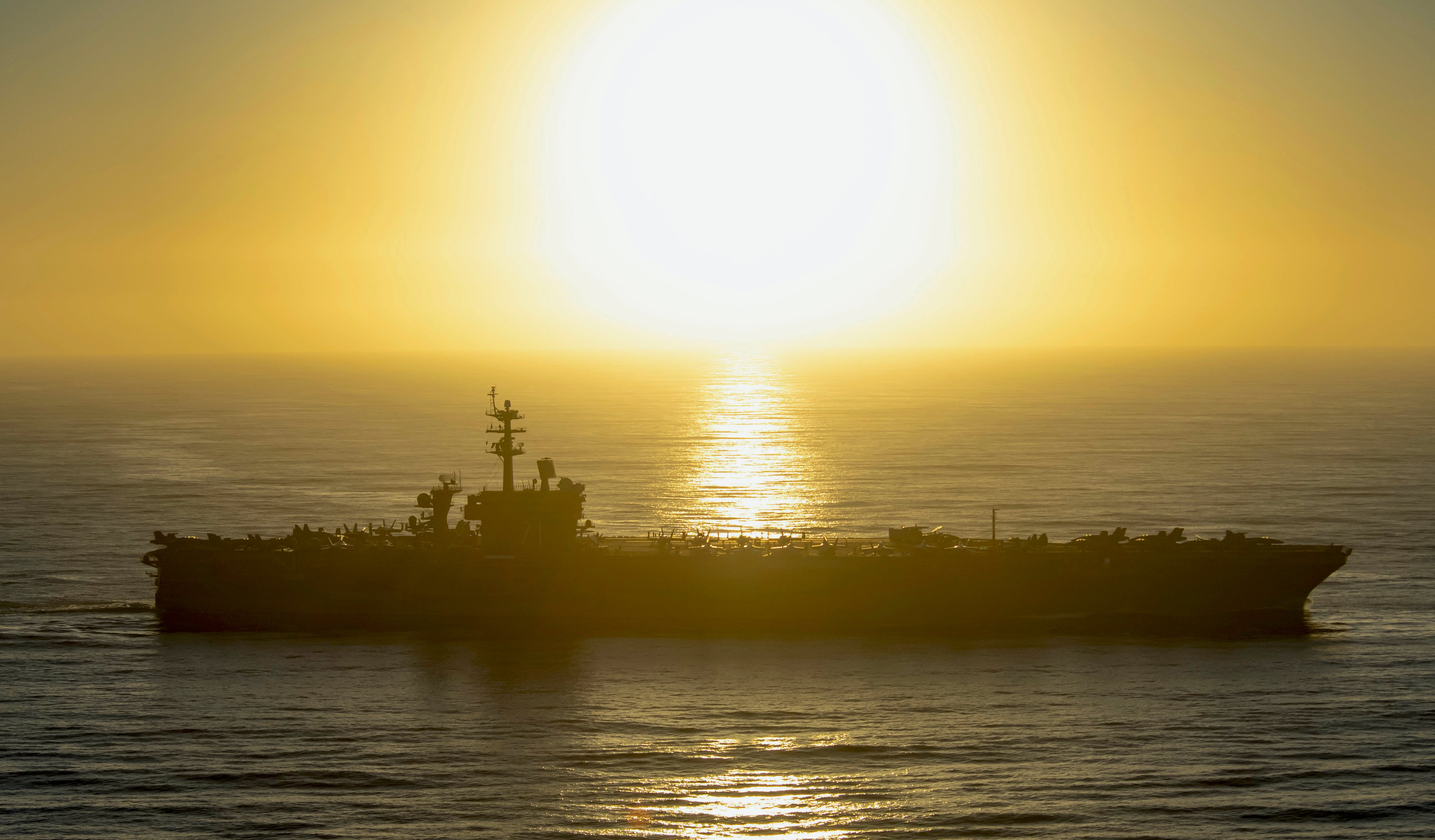In this evocative image, a large aircraft carrier, possibly a military warship, is silhouetted against a breathtaking sunrise or sunset. The sky is a brilliant orange hue, with a large, white circular sun at the center. The sun's light creates a dazzling path of reflection across the calm, rippled ocean, extending from the horizon well into the foreground. The water, predominantly dark bluish-gray, contrasts starkly with the sun's luminous reflection. The ship itself is depicted mostly in dark outline, stretching almost the entire width of the image. The deck of the vessel is cluttered with various pieces of equipment and what appear to be planes positioned both at the front and back. A prominent mast is visible towards the left side. The scene exudes a peaceful yet powerful atmosphere, heightened by the serene, ripple-textured sea and the striking visual pathway of light emanating from the sun.